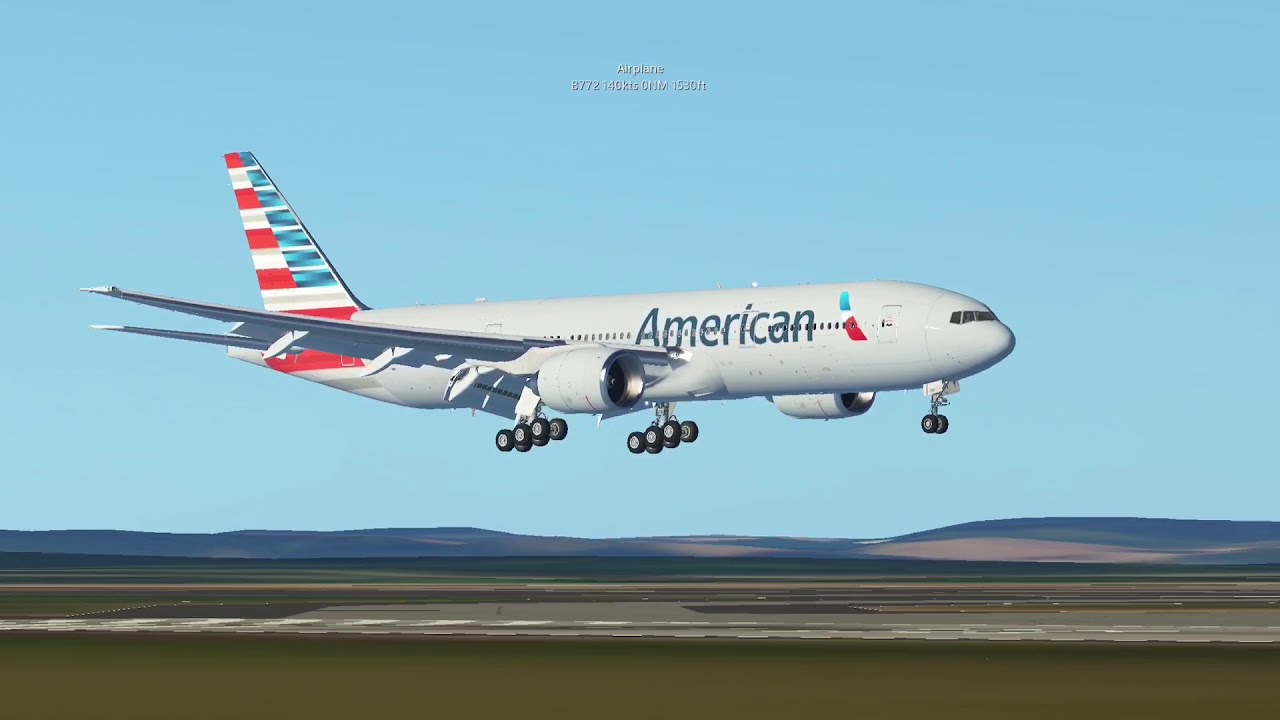This image depicts a computer-generated scene of an American Airlines jet airplane, likely a Boeing 737, either landing or taking off on a runway. The airplane is a large, white aircraft with the word "American" emblazoned in blue on its forward fuselage and adorned with the iconic American eagle logo in red, white, and blue. The tail fin features an alternating pattern of red, white, and blue rectangles. The jet is shown in profile, facing right, against a backdrop of a bright, cloudless blue sky. The landing gears are fully extended, with two rows of four wheels each under the main body and standard two-wheel nose gear. Below the aircraft, the landscape comprises a realistic-looking flat, smooth, rising hillside and a grassy area leading up to the paved asphalt runway, suggesting this could also be part of a video game scenario. The attention to detail in both the airplane and the surrounding environment adds depth and realism to the image.